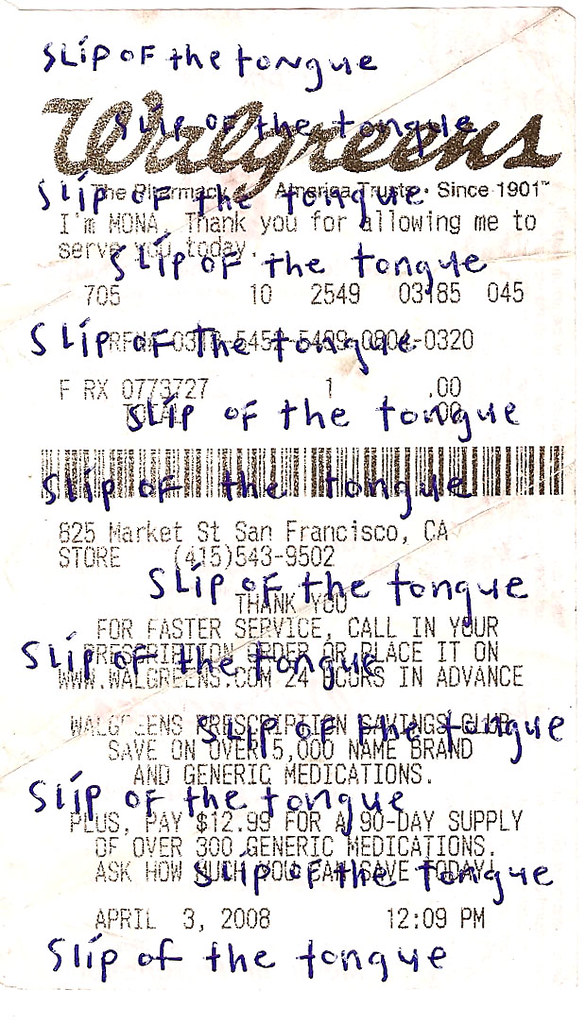The image is an overexposed photo of a Walgreens pharmacy and convenience store receipt, rendering the paper almost pure white with minimal visible texture. Despite the overexposure, the receipt shows minor signs of wear including subtle creases and small dirt marks scattered across it. A prominent barcode is located in the middle of the receipt, and directly below it, text indicates that the purchase was made at a Walgreens on Market Street in San Francisco, California. The receipt has been transformed into a visual collage, featuring numerous handwritten lines in pen. Each line repeats the phrase "slip of the tongue" approximately ten times from the top to the bottom of the receipt.